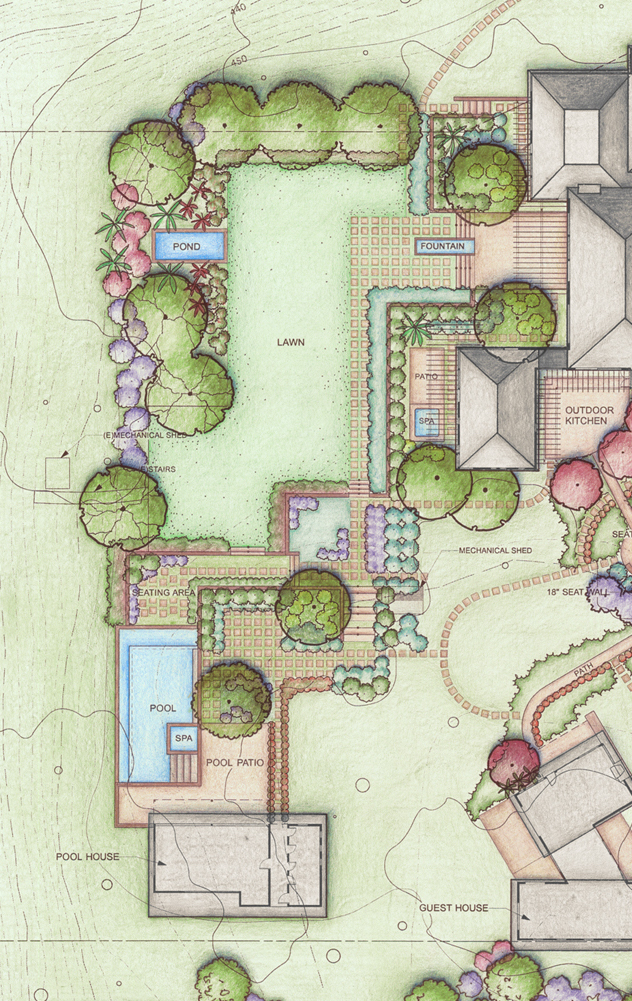The image depicts a detailed bird's eye view of what appears to be a resort or a luxurious residential property, showcasing a variety of well-labeled structures and lush vegetation. The background of the map is predominantly green, indicative of the abundant trees and plants throughout the area. Key features include a pond situated in the upper left corner, surrounded by bushes. Adjacent to it, in the lower left section, is a rectangular pool accompanied by a square spa. This area also features a pool patio with a designated seating area. Directly below the pool is the pool house. 

On the upper right side of the map, there is a fountain, while the middle right side is designated for the outdoor kitchen, which is characterized by a reddish lettering. The central area, likely representing the main house, includes pathways and additional labeled sections such as lawn, patio, and spa. Towards the bottom right-hand corner is an arrow pointing to the guest house. The landscape is intricately detailed with approximately twelve bushes scattered across the lawn, enhancing the verdant aesthetic of the property.